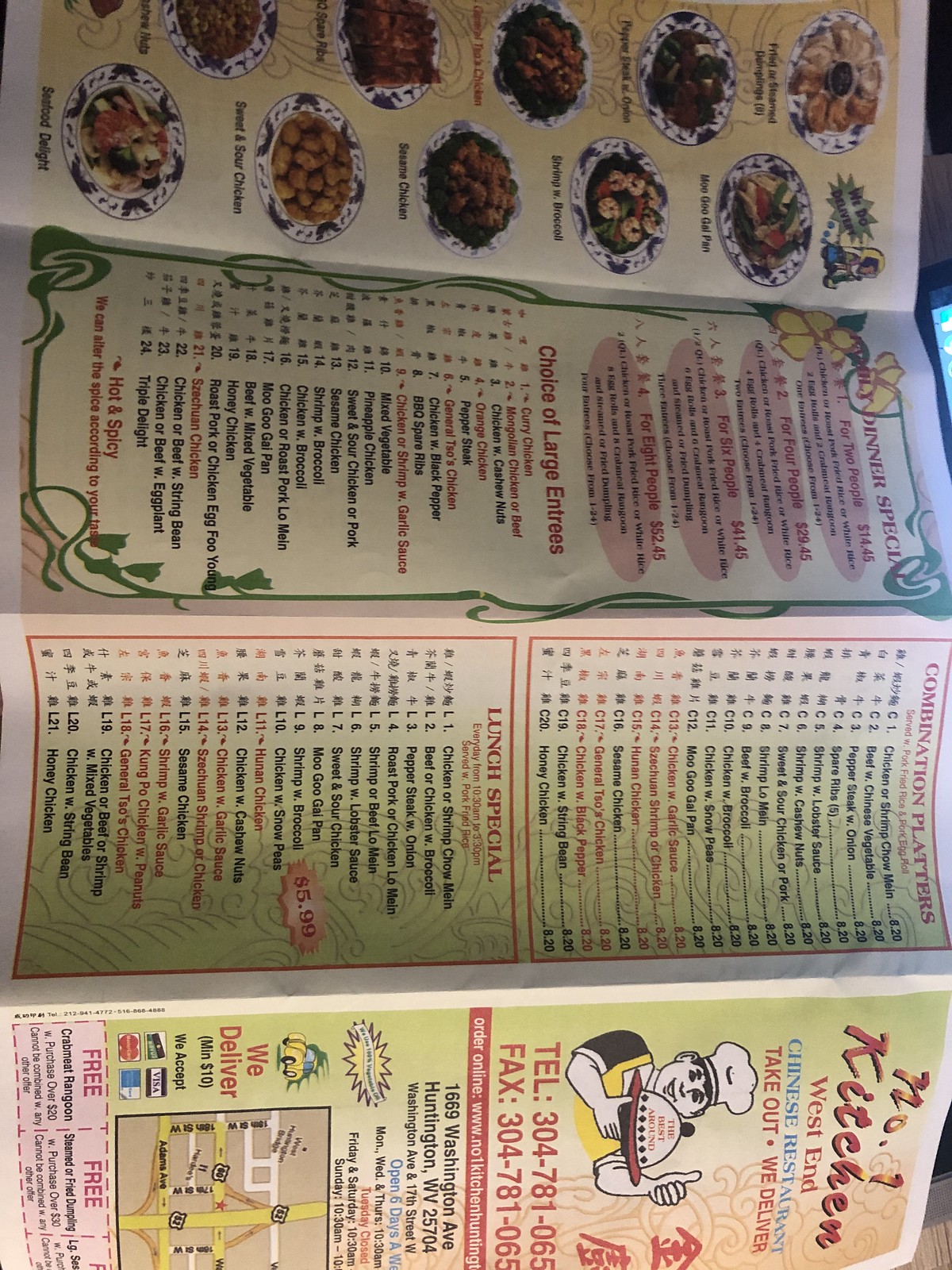The photograph captures a Chinese takeout menu, unfolded and consisting of four sections. The image is oriented such that the top of the menu is rotated to the right, while the bottom faces downwards. Despite being slightly blurry, several details are discernible. 

At the top of the image, two vertical rows each display five photographs of various dishes, showcasing vibrant plates of food. The next section, listing large entrees, includes an array of itemized choices, but the font is too small to decipher the exact entries and their corresponding prices. Moving further, another section appears with additional options listed, yet again, these details are unreadable due to the small font size. 

The bottom part prominently features lunch specials, leading down to the very bottom of the image where the front cover of the menu is displayed. This cover includes an illustration of a person wearing a chef's hat and holding a plate with a lid, hinting at the culinary delights within.